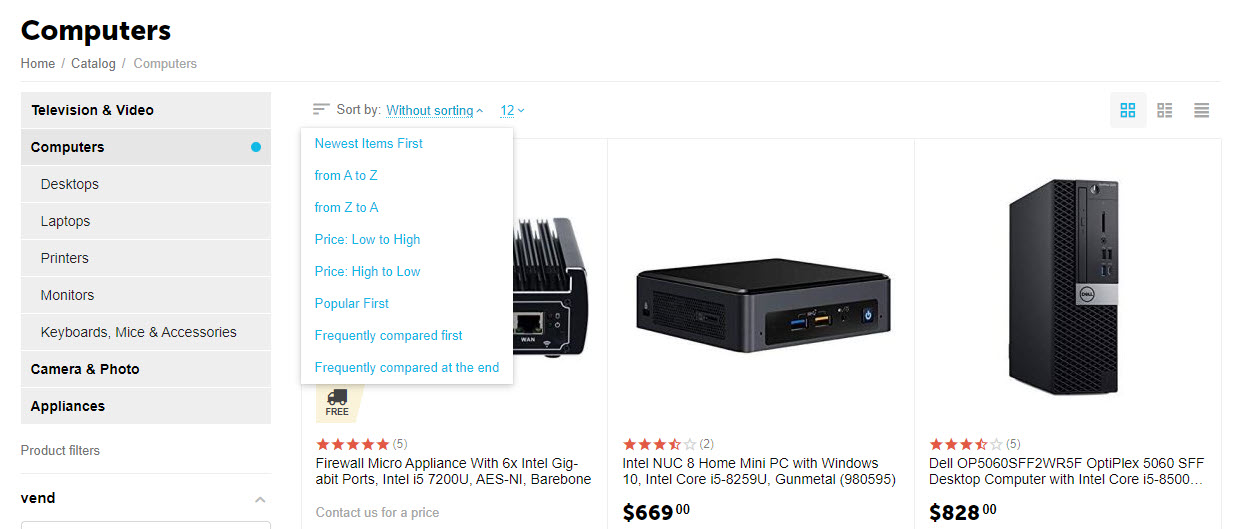This is an online retail website featuring a detailed catalog section for computer-related products. The left sidebar begins with a header labeled "Computers" and a breadcrumb navigation indicating "Home / Catalog / Computers." Below this, there's an organized list of product subcategories. The primary category displayed is "Television and Video," with "Computers" as a secondary focus. Under the Computers subcategory, there are further divisions including "Desktop," "Laptop," "Printers," "Monitors," "Keyboards," "Mice," and "Accessories."

Continuing down the sidebar, additional main topics of interest include "Camera and Photo," "Appliances," "Product Filters," and "Vend." The site features an expandable menu section for sorting options, offering choices such as "Sort By," "Without Sorting," "Newest Items First," "From A to Z," "From Z to A," "Price Low to High," "Price High to Low," "Popular First," and "Frequently Compared First."

Displayed prominently on the main section of the page are three featured product listings. The first product is a "Firewall Micro Appliance with 6x Intel Gigabit Ethernet." The second is an "Intel NUC and Home Mini PC with Windows." The third item is a "Dell OptiFlex 5060SFF Desktop Computer with Intel Core." Each product is accompanied by relevant specifications and differentiating features.